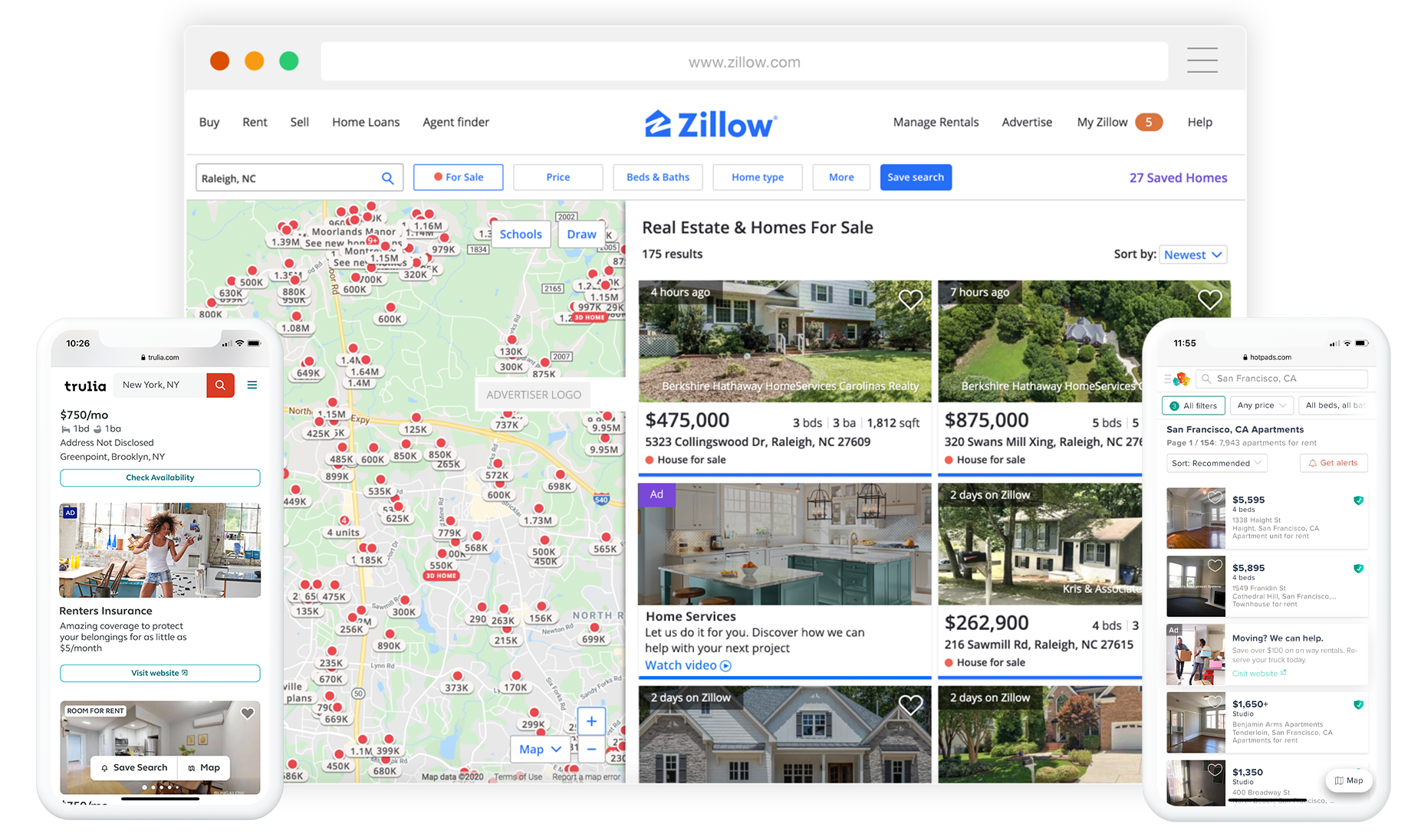A detailed caption for the image:

This image is a composite screenshot featuring the Zillow application on various devices. The central screenshot, displayed on a widescreen tablet or laptop, showcases the main Zillow interface. Here, you can see a grid with six property listings, arranged in two columns and three rows, each displaying an image, price, and address of homes located in Raleigh, North Carolina. To the left of the property listings, there is an integrated map resembling a Google map, pinpointing additional properties for sale in the area with red circles indicating their locations and price tags.

Flanking the central screenshot are two narrower, vertically aligned screenshots, likely from iPhone devices. These are overlaid on the left and right edges of the central image. Both of these side screenshots exhibit other sections of the Zillow app, focusing on different property listings with images and prices prominently displayed.

All elements across the screenshots highlight the Zillow brand, identifiable by its signature blue house icon with a stylized 'Z' and accompanying "Zillow" text.